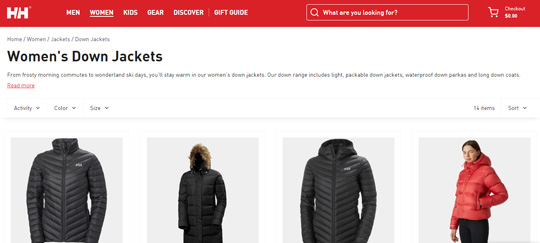The image depicts a webpage from Helly Hansen's online store, showcasing their collection of women's jackets. The webpage is themed in a red and white color scheme, with white text on a red background.

At the top left of the page is Helly Hansen's logo, represented by a white "HH" with a distinctive horizontal gap between the two "H"s. To the right, there is a navigation bar allowing users to shop for men’s, women’s, and kids' gear, explore the discovery section, and view the gift guide. An emphasized section for women’s products is highlighted to the right. A search bar is available along with a shopping cart icon displaying a "$0" balance, indicating no items have been added.

On the left sidebar, a breadcrumb navigation starts with "Home," followed by categories "Women's Jackets" and "Down Jackets," allowing users to refine their selection further. Four product images are prominently displayed. 

1. The first jacket, modeled, is a full-zip, horizontally ribbed design with white branding on the left breast.
2. The second jacket features a furry hood.
3. The third jacket, similar to the first, extends slightly higher for a turtleneck effect and is also ribbed.
4. The fourth is a puffy hooded jacket modeled by a woman with her left hand in her pocket.

Above these images is a dropdown menu for selecting color and size, and a link for additional information about women’s jackets. Although the page indicates that there are 14 jacket options, only four images are shown in this snapshot.